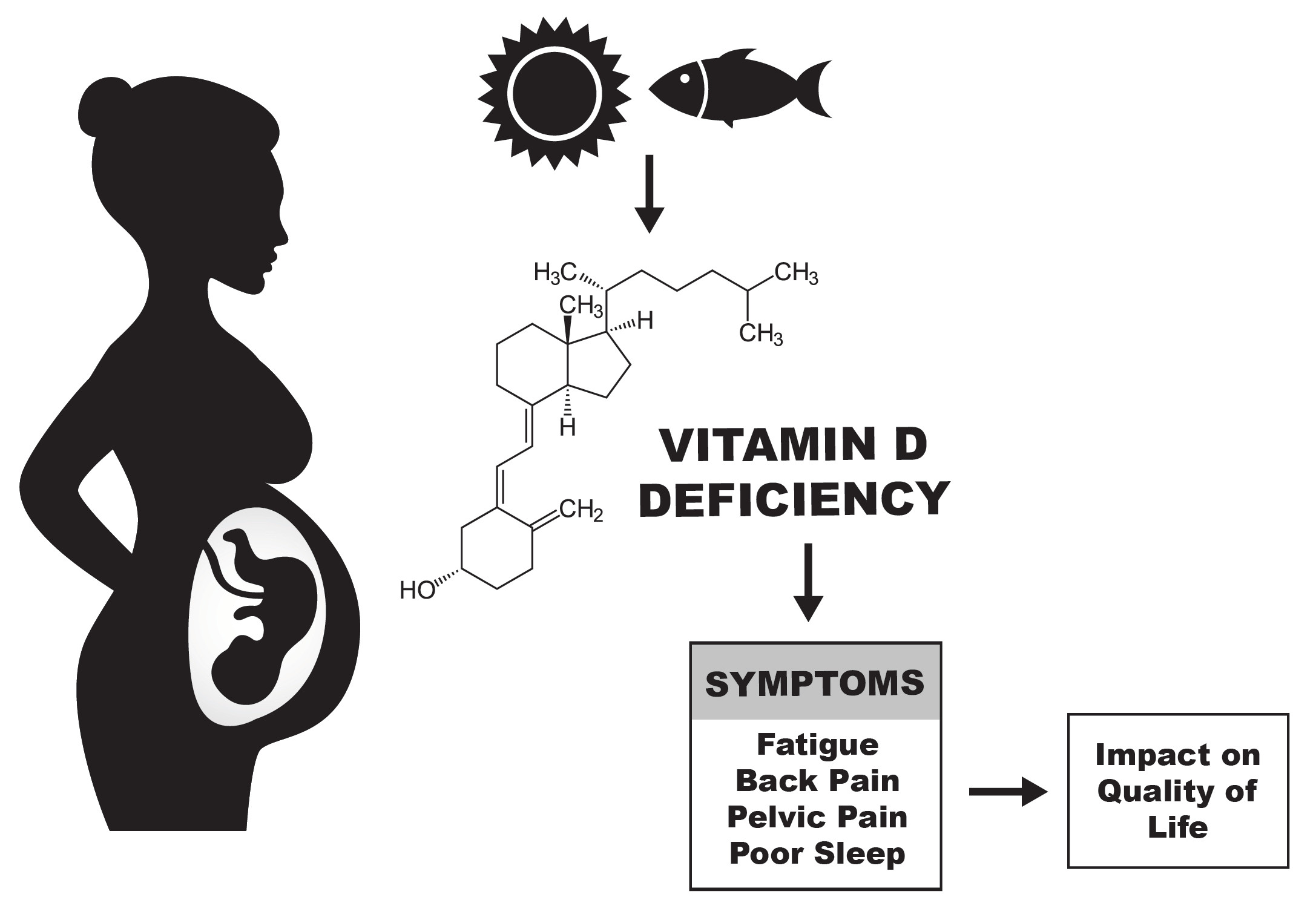The informational poster for pregnant women suffering from vitamin D deficiency features a clean black-and-white design on a white background. On the left side, there's a black silhouette of a pregnant woman with her hand on her hip and hair in a bun. Visible inside her belly is a white oval shape depicting a fetus. Above the silhouette, there's a black icon of a sun and a fish, both pointing down towards a detailed molecular structure of vitamin D, showcasing compounds such as HO, CH2, H, CH3, H3C, and CH3. Below this structure, bold black text reads "Vitamin D Deficiency," leading to an arrow pointing down to a box with a gray border listing symptoms: fatigue, back pain, pelvic pain, and poor sleep. An arrow from the symptoms box points right to another box with a black border, detailing the impact on quality of life.